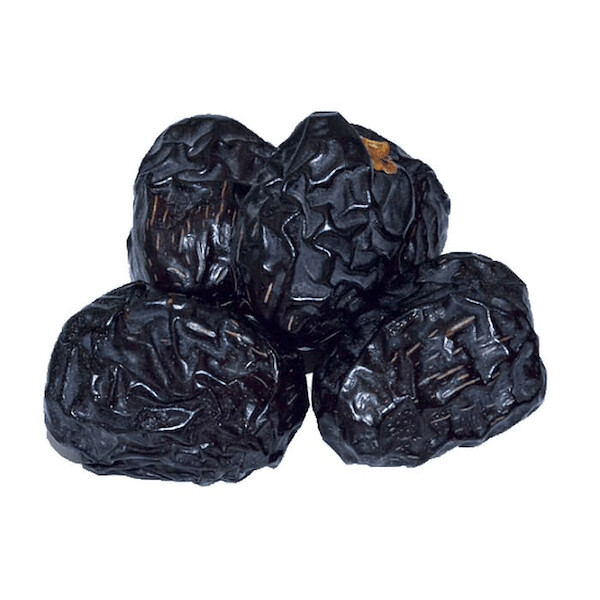This is a detailed photograph of four dried pieces of fruit, identified as prunes due to their dark bluish-black to purple hue. The image features a clean, stark white background, enhancing the contrast and clarity of the prunes. The four prunes vary slightly in their arrangement: two are lying flat on their sides, one is propped up vertically, and they form a small stack. Each prune exhibits substantial wrinkling, indicative of their dried state, with occasional glistening spots suggesting residual stickiness and a once-shiny skin. A notable detail is the small brown stem on the prune positioned on top, adding a touch of natural texture to the otherwise dark and shriveled appearance of the fruit.